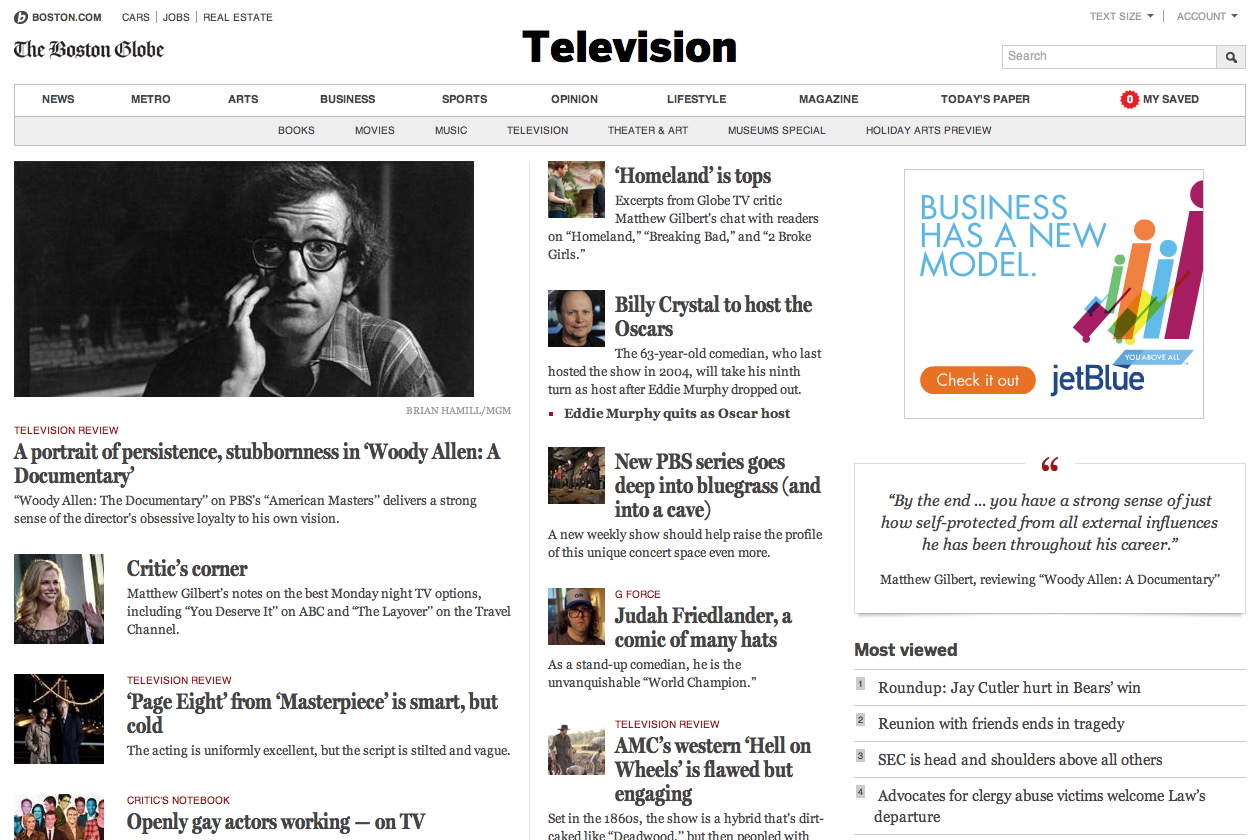The homepage of The Boston Globe is prominently displayed, featuring their distinctive cursive logo at the top. Above the logo are links to related sections: Boston.com, Cars, Jobs, and Real Estate. Central to the page is a prominent "Television" header. A search box adorned with a black magnifying glass icon is easily noticeable, allowing users to search the site. 

The page is neatly organized into various sections, including News, Metro, Arts, Business, Sports, Opinion, Lifestyle, Magazine, Today's Paper, and a 'My Saved' section for personalized content. Beneath these categories, a diverse array of articles and images provides engaging content for readers.

The lead article, titled "Television Review: A Portrait of Persistence, Stubbornness, and Woody Allen," features a documentary on Woody Allen as part of PBS's American Masters series. This piece is accompanied by an image of a man wearing black glasses, emphasizing Allen's unwavering dedication to his artistic vision.

Another highlighted piece is "Homeland is Tops," which includes expert opinions from Globe TV critic Matthew Gilbert. This article offers insights into popular TV shows such as "Homeland," "Breaking Bad," and "Two Broke Girls." 

Additionally, in "Critic's Corner," Matthew Gilbert provides notes on the best Monday night TV options, spotlighting shows like "You Deserve It" on ABC and "The Layover" on the Travel Channel. This article is visually supported by an image of a blonde woman waving, donned in a black dress. The overall aesthetic of the page includes mostly black text set against a clean white background, ensuring readability and a pleasing visual experience.